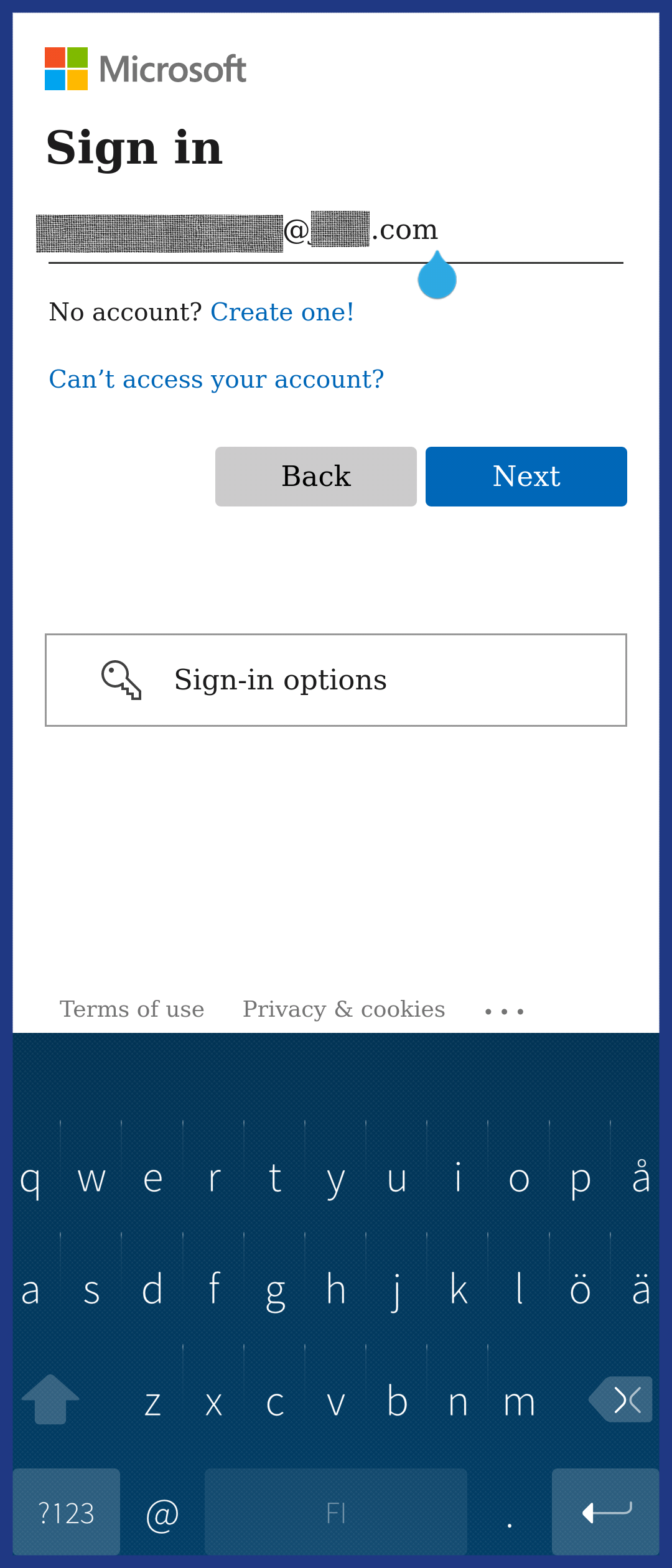This image is a screenshot taken from a mobile phone, as indicated by the tall rectangular frame and the visible QWERTY keyboard at the bottom for typing. The screenshot is bordered by a thin blue line, complementing the bluish tone of the keyboard area. The main content of the screenshot features a white background displaying the Microsoft Hotmail sign-in page.

At the top of the page, the Microsoft logo is clearly visible. Below it, there's the Hotmail or email sign-in form that reads "Sign in," but the specific email address has been redacted. The redaction appears to be a piece of tape covering the address, with only the "@" and ".com" visible. 

Further down, the page displays typical options such as "No account? Create one!", "Can't access your account?" followed by a question mark. Two buttons labeled "Back" and "Next" are positioned underneath these options. At the bottom of the screenshot, there is a "Sign-in options" link accompanied by a key icon.